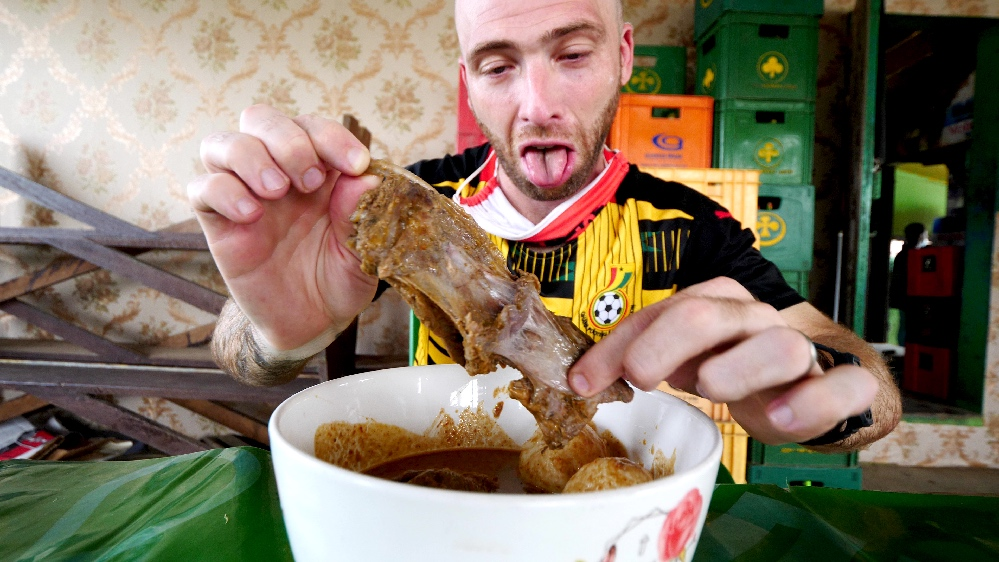This photograph captures a man sitting at a table covered with a green tablecloth, engaged in the act of peeling meat from a bone with both hands. The dish he hovers over is a white bowl containing what appears to be a hearty beef stew, with visible chunks of meat, possibly potatoes, and a red sauce. He wears a multicolored soccer jersey featuring a soccer ball emblem on the chest, comprising hues of black, yellow, green, and red. The man has a beard and a mustache, and while the top of his head is obscured, he seems to be bald. His facial expression displays a mix of intrigue and possible disgust as his tongue sticks out, seemingly about to take a bite or perhaps hesitant about the taste.

The setting is inside a somewhat cluttered interior space that appears informal and a bit mismatched. Behind him, the wall sports a formal golden design wallpaper, although some describe it as cream-colored. There are numerous crates and boxes stacked against the wall in various colors, including green, orange, yellow, blue, and red. A park bench-like structure is also leaning against the wall. Through an open green door in the background, one or two blurred figures can be seen in another room, adding to the incongruence of the scene. The room's ambiance suggests a place not typically used for dining, adding an element of curiosity to the photograph.